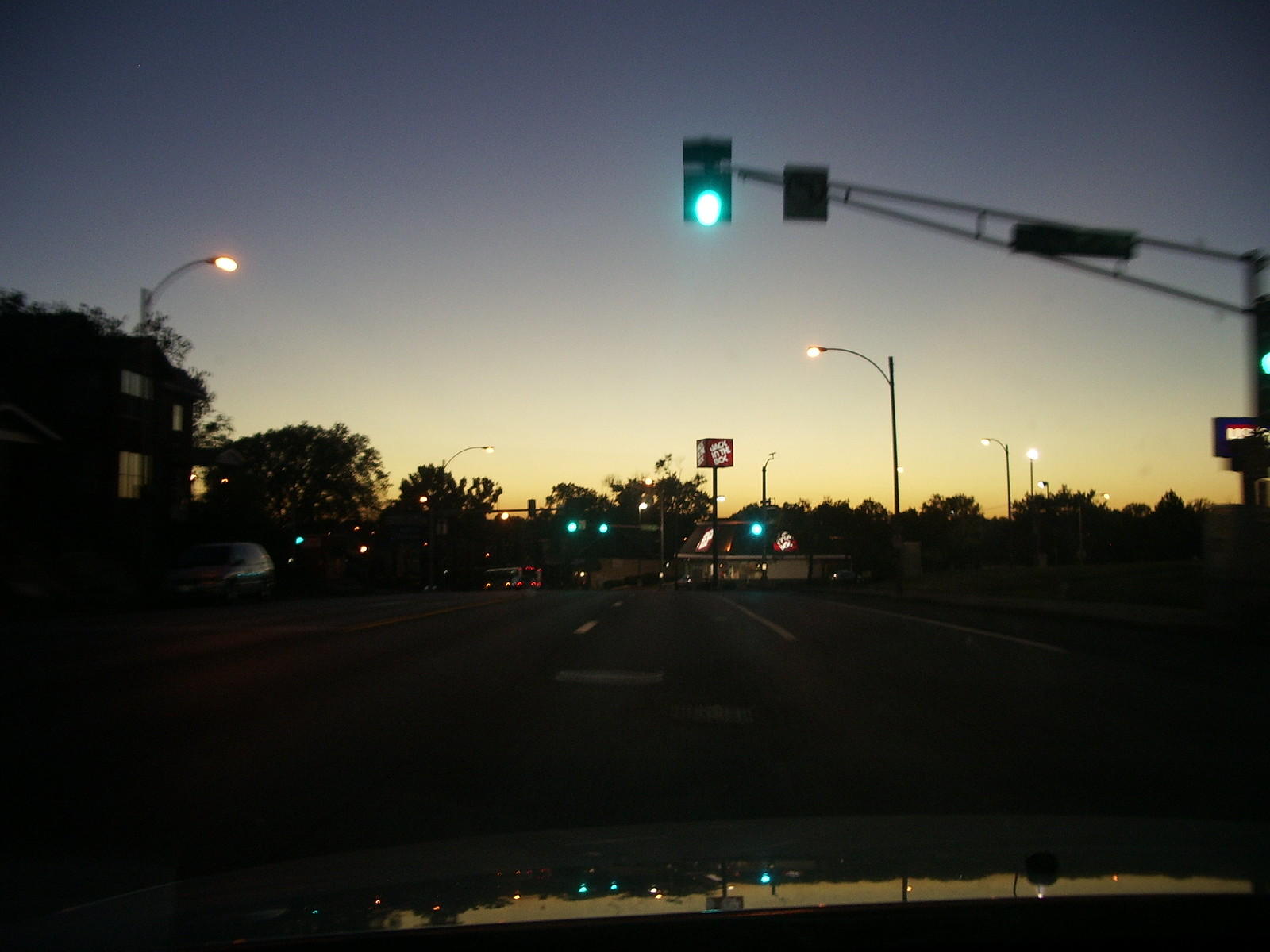This color photograph, taken at night through the windshield of a vehicle, depicts a city street under a beautifully gradient sky transitioning from a purple-blue at the top to a light yellow at the horizon. The majority of the image is underexposed, adding to the nighttime ambiance. In the foreground, reflections and shine from streetlights and traffic lights appear on the vehicle's hood, suggesting the photo was taken from inside a moving car.

Central to the scene is a roadway with white broken lane markings leading into the distance. A green traffic light hangs from a steel gantry on the right side of the image. On the left side, a shadowy building can be seen with illuminated glass window panes. In the distance on the right side, a Jack in the Box fast food restaurant is visible, identifiable by its illuminated red square sign and an advertising cube on a tall pole. This sign is designed to be seen from multiple directions. Trees and additional streetlights dot the background, adding depth to the urban setting. There are also a few distant cars near the restaurant, reinforcing the night-time cityscape atmosphere.